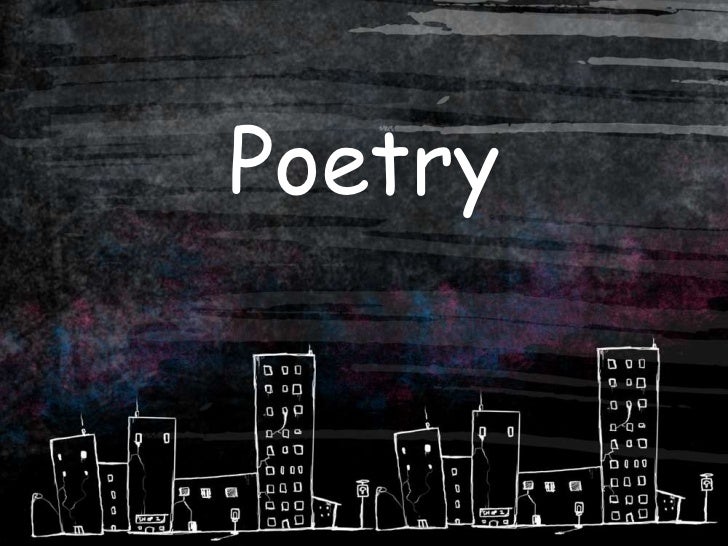This image is a detailed black-and-white drawing featuring a cityscape, set against a dark background that appears to be painted with a black stain, allowing the wood grain to subtly show through. At the top of the image, the word "Poetry" is prominently displayed in thick, white font. Below this text, the hand-drawn cityscape unfolds, depicting various downtown buildings of different heights. These buildings are filled with numerous little square windows, indicating large apartment structures. The cityscape also includes intricate details such as stop signs and street lights along the route, enhancing the urban feel. The structures, drawn in white pencil, appear slightly sloppy, reminiscent of a child’s drawing, adding a charmingly imperfect quality. Some buildings are tall with seven or eight rows of windows in a three-across pattern, and one on the far right even features a garage. A couple of street signs punctuate the scene, and there’s a quirky building that tilts slightly, giving the impression of a quaint, bustling city. The overall style suggests it could serve as the cover for a poetry book or picture book.